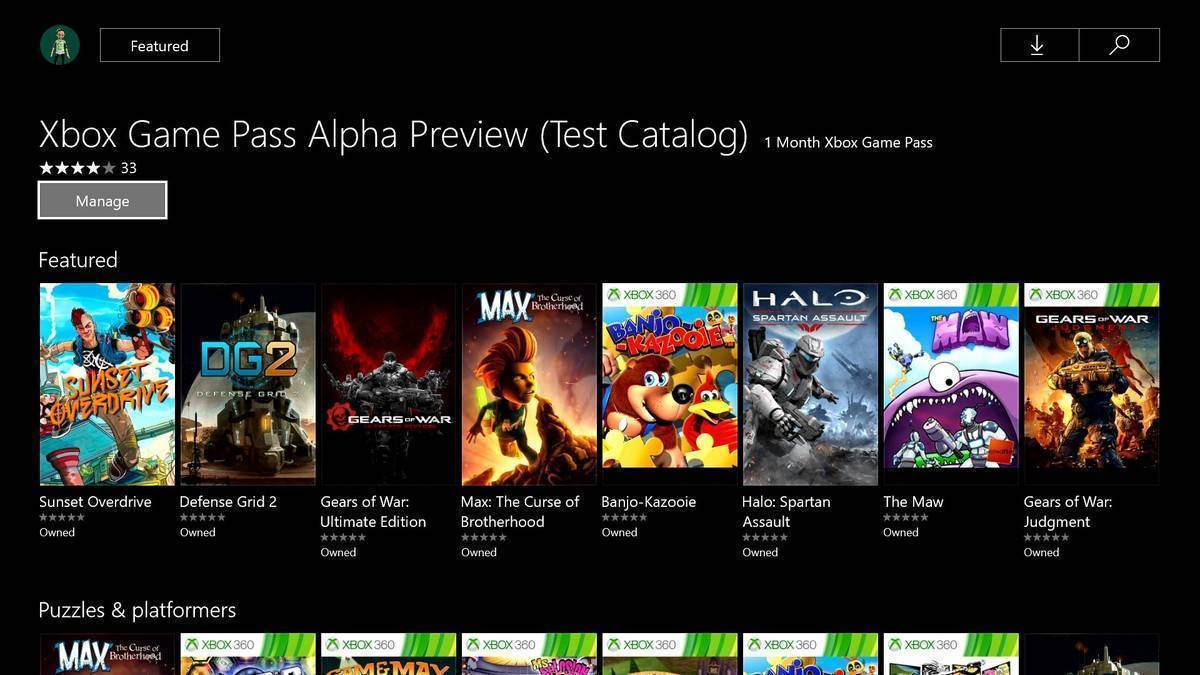This is a detailed caption for an image of an Xbox Game Pass catalog interface:

---

The image is a screenshot of the Xbox Game Pass catalog featuring a dark or black background. On the top left, there is a user profile photo depicting a game character. To the right of the profile photo is a rectangular section where it reads "Xbox Game Pass Alpha Preview" with "test catalog" in brackets. Adjacent to the text, a small line of text details "one month Xbox Game Pass."

To the top right, flanking the catalog title, are a search button symbolized by a magnifying glass and a download button. Below this, the interface displays a rating of four out of five stars based on 33 ratings. There is also a gray "Manage" button with white text and a white border.

The featured games are displayed in a grid below this section, including titles like "Sunset Overdrive," "Defense Grid 2," "Gears of War: Ultimate Edition," "Max: The Curse of Brotherhood," "Kameo: Elements of Power," "Halo: Spartan Assault," "The Maw," and "Gears of War: Judgment." All games are marked as owned and display five gray stars indicating no actual rating. Each game is represented with their colorful cover art, some showcasing the Xbox 360 logo which resembles the actual physical game boxes, while others are represented with graphics.

Below the featured section, there is a partially visible row labeled "Puzzles and Platformers," with additional game images that are only partially within the frame, about 15% cut off from the bottom.

---

This caption offers a clear and intricate description of the screenshot, helping readers visualize the layout and contents of the Xbox Game Pass catalog interface.